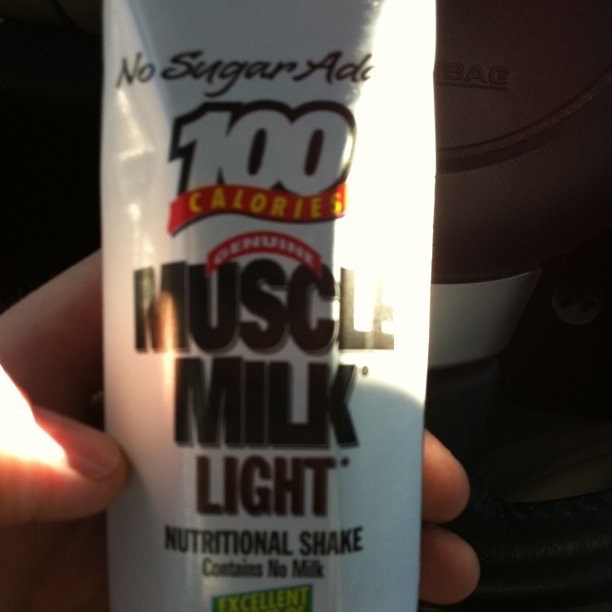The image depicts a left hand with pudgy fingers and short nails holding up a white rectangular package of "Genuine Muscle Milk Light Nutritional Shake" in the passenger side of a vehicle, as indicated by the visible airbag. The package prominently features the text "No Sugar Added" at the top in brown, and "100 Calories" below it with the number '100' outlined in brown and white, and 'calories' in yellow on a red ribbon background. The largest font on the packaging reads "Muscle Milk" in dark brown, with "Light" below it in light brown. The nutritional claims, including "Contains No Milk" and "Nutritional Shake," are in black text. An "Excellent" green tag with yellow lettering is also visible at the bottom. The background of the image is mostly white with some visible areas of red and green details on the package.